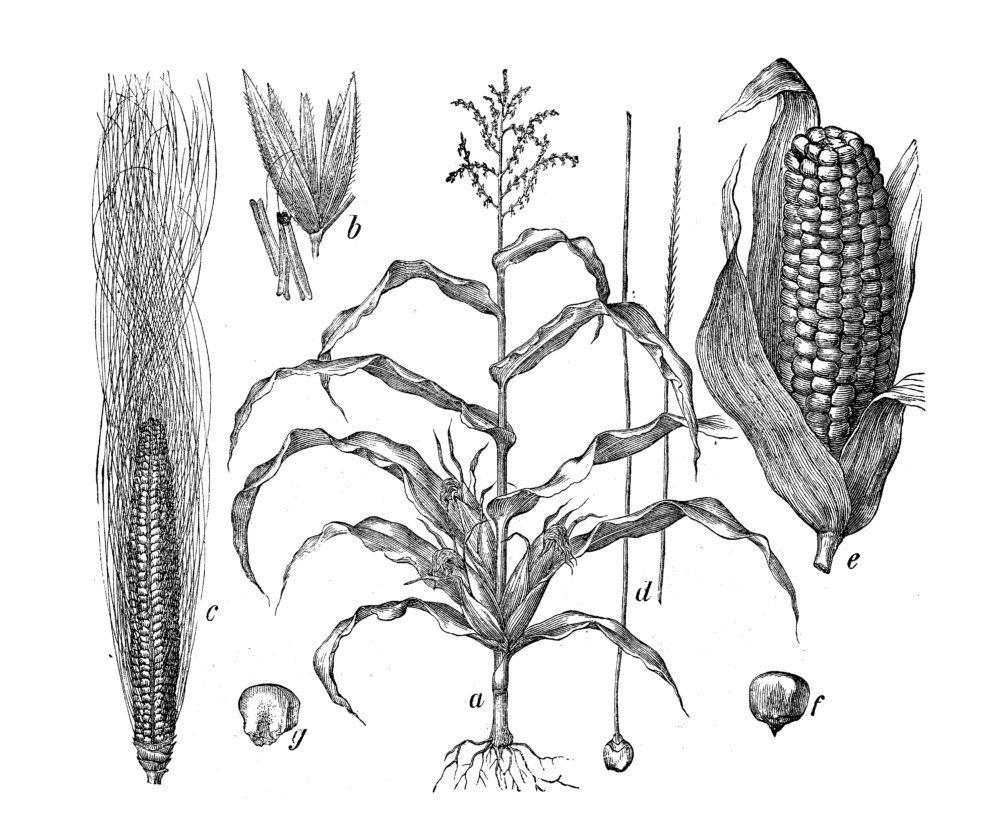The black and white hand-drawn image is a detailed diagram of various stages and parts of a corn plant labeled from A through G. Positioned on the left side is a long, peeled corn cob with extensive fine strands labeled 'C,' stretching from the head at the bottom left upward and almost reaching the top right of the image. In the center, there is a thin-stalked corn plant with numerous alternating slender and curved leaves, and visible roots at the bottom of the stalk, along with corn cobs growing about a quarter from the bottom of the plant. This central plant is labeled 'A.' 

On the right side, there is a regular corn cob with its husk partly peeled back, labeled 'E.' Additionally, the image includes detailed depictions of individual corn kernels in various growth stages, labeled 'F' and 'G,' alongside a magnified image of fine filaments and pollen structures labeled 'B.' Below the central corn plant, a small, sprouting corn seed labeled 'D' can be seen, illustrating the plant's developmental process. This comprehensive diagram offers an etched visualization of corn's physical structure and different growth phases.